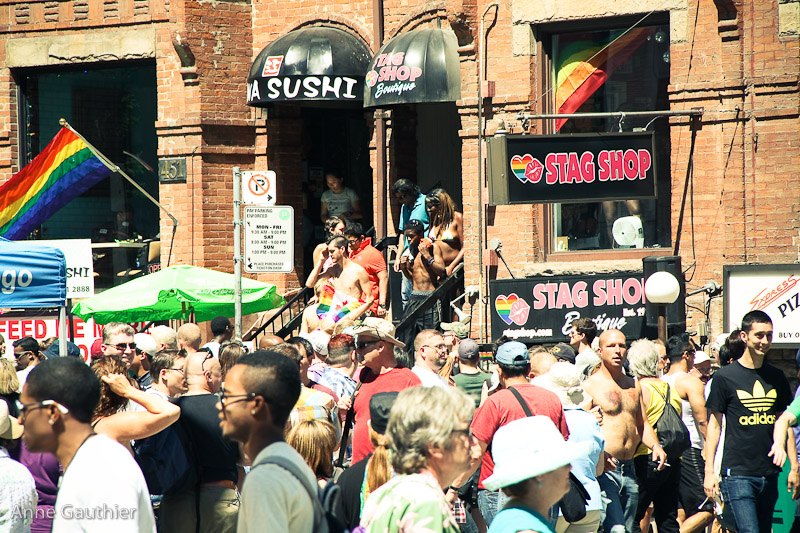The photograph captures a bustling scene of a large crowd gathered on a sunny day in front of a series of red-orange brick buildings lining a street. Prominently featured are two storefronts with awnings; the left one bears the word "Sushi" in white font, while the right one reads "Stag Shop" in bold red letters. Additionally, the "Stag Shop" name appears again on a hanging sign affixed to a pole jutting out from the building. There are vivid green umbrellas set up near the stores, offering some shade. A pride flag is visible on the left side of the image, adding to the festive atmosphere. The diverse crowd includes several shirtless individuals, indicating the warm weather. A no parking sign is situated on a metal pole in the foreground. The scene suggests an event or parade, as people enjoy the sunny day and the lively surroundings.